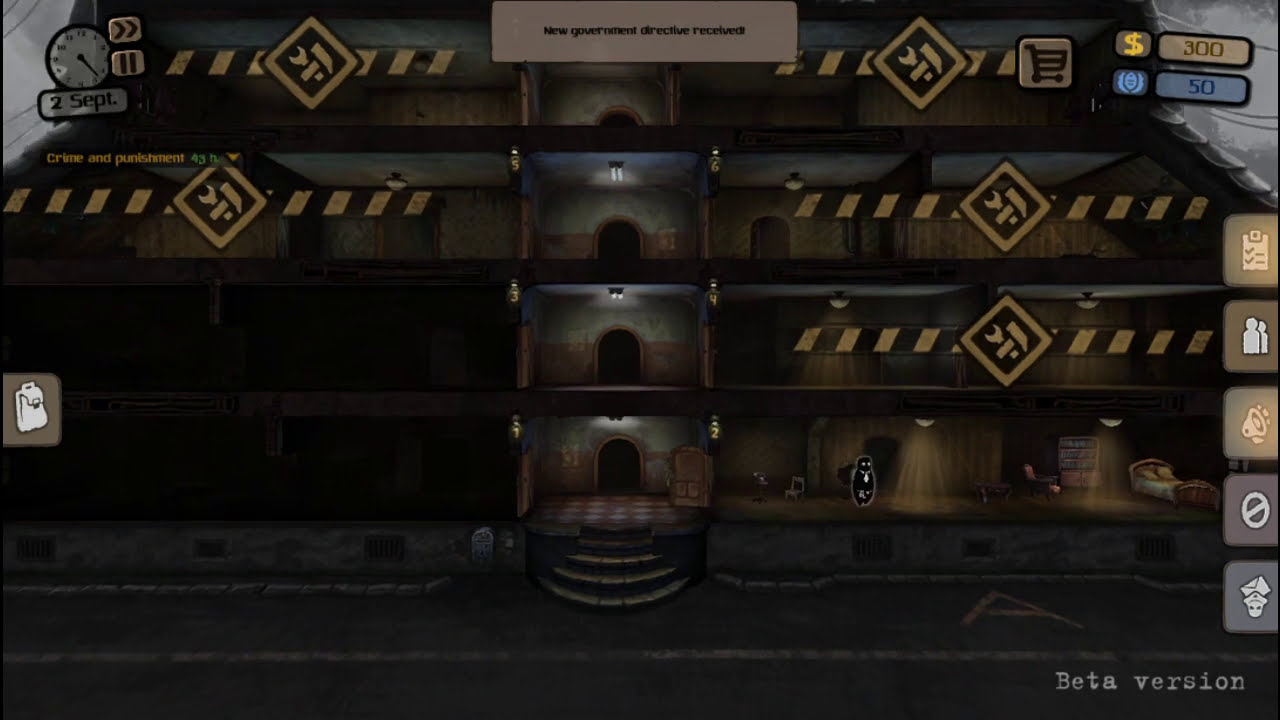The screenshot depicts a dark and gloomy video game set in what appears to be a large, old, beat-up house or apartment building, which resembles a haunted castle under construction. The building spans multiple floors, each with various doors and pathways. The lower floor, where the player character is currently located, is dimly lit, while the floors above remain largely in darkness, suggesting they are under construction with construction tape marking areas the player cannot access yet. At the top of the screen, the message "New government directive received" is displayed, accompanied by various symbols including a clipboard, a friends icon, and a megaphone. The street in the foreground features a solid white line and the overall scene appears to be quite intricate with detailed graphics. The bottom right corner of the screen indicates that this is a "beta version" of the game. On the game's interface, five squares host different icons like a loud horn, a speaker, and a checklist, presumably for various in-game functionalities. The detailed structure of the building and its maze-like quality enhance the complexity and eerie atmosphere of the game.